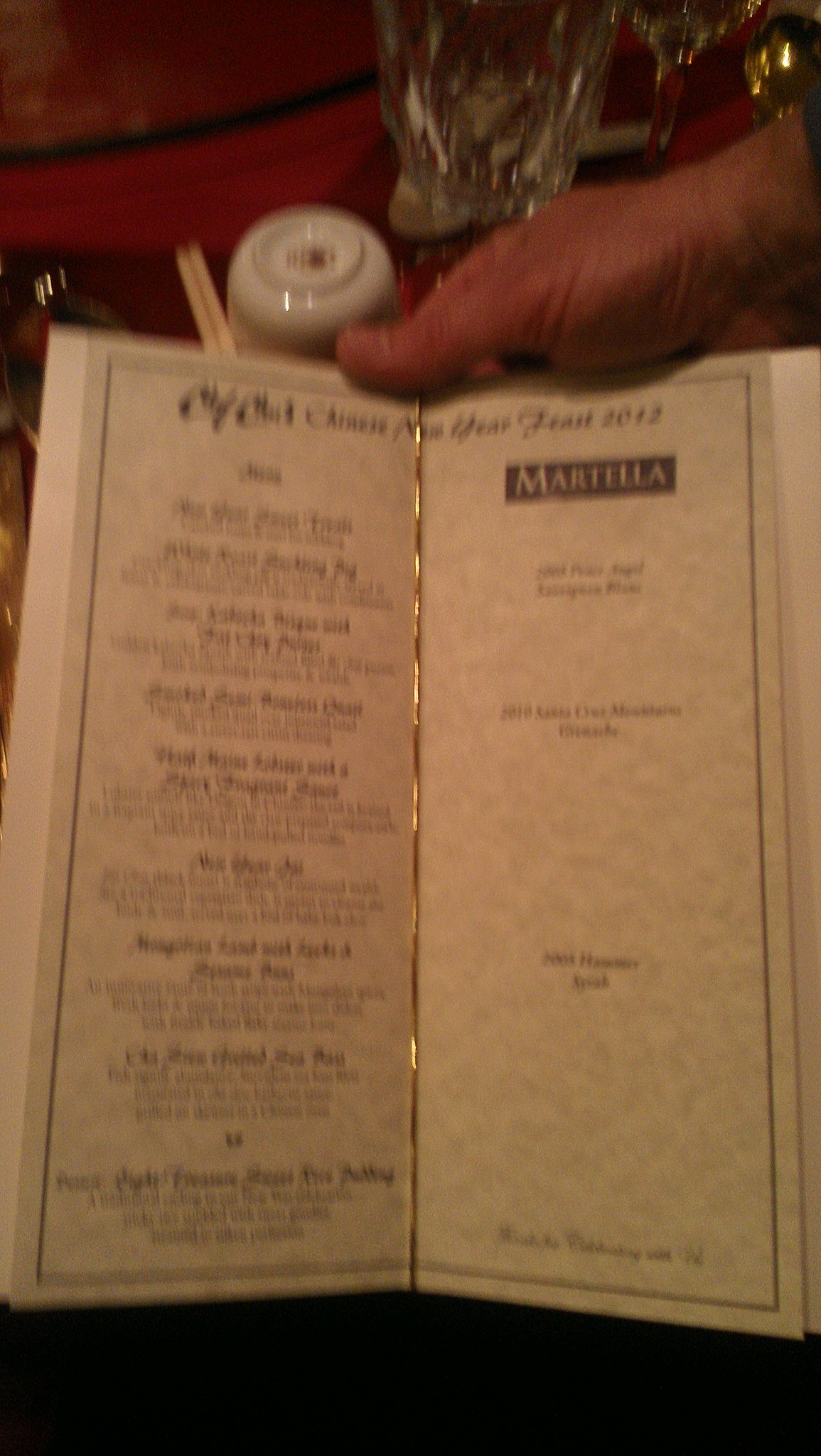A person holds a tan booklet, possibly a menu or program, with a white border while taking a photo with their left hand. The photo, though blurry and of poor quality, captures the detailed layout of the items on the booklet. The person’s hand is prominently placed over the top of the booklet. The title “FEAST 2012” is partially visible at the end of the booklet, suggesting it pertains to an event or dining experience from that year. The left side of the booklet lists approximately nine items each with detailed descriptions, reinforcing the idea that it is likely a menu or program. On the right side of the booklet, a rectangular brown box with white text spells out "MARTILLA," with three spaced-out lines of text beneath it. Above the person's hand is a white coffee cup with blue trim, set next to a glass pitcher of water. The objects are arranged on a red placemat atop a wooden table, providing a contextual background for the scene.